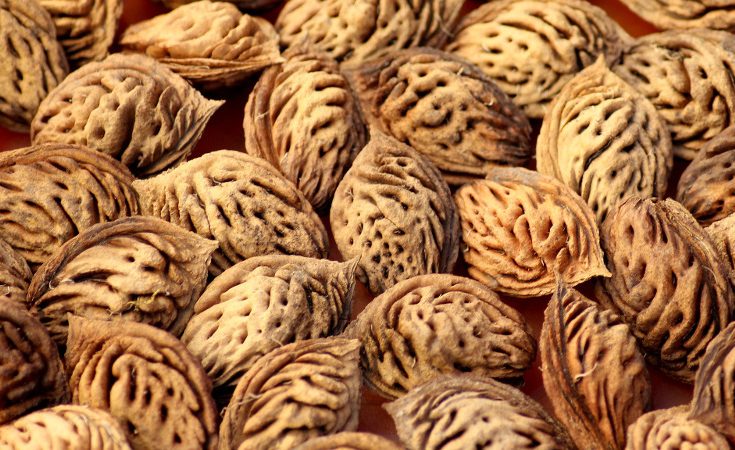This image captures a close-up landscape of around 20 to 30 fruit pits, likely from peaches or nectarines, although some might mistake them for walnuts due to their intricate, textured surfaces. The pits, varying in shades from light tan to dark brown, are scattered across a reddish-brown background that resembles a wooden table. The natural light hits the scene from a top-down angle, highlighting the fibrous texture and deep, dark crevices of the pits, which create striking shadows and depth. The tips of the pits are pointed, adding to their rugged appearance. This detailed composition focuses solely on the fruit pits, devoid of any additional elements or text.